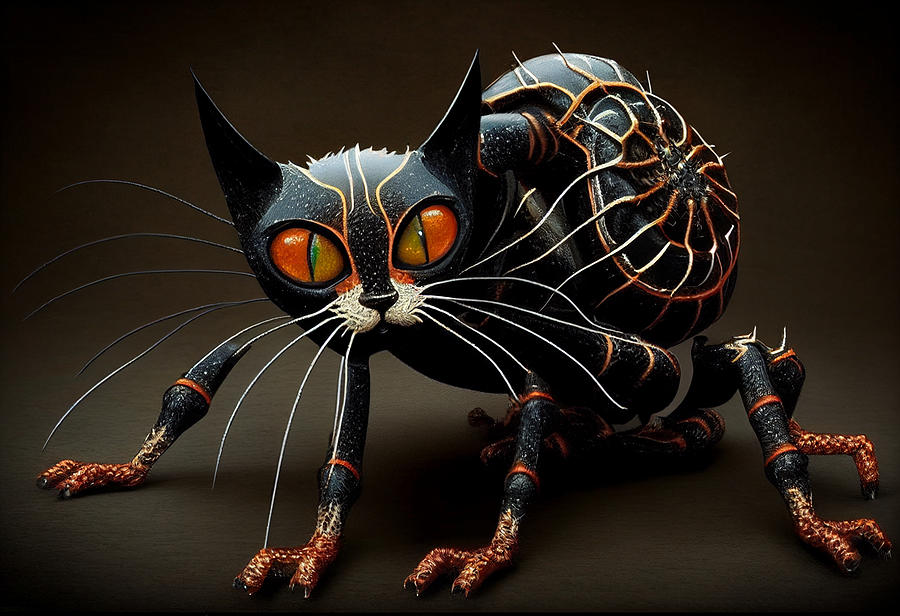This detailed horizontal rectangular image, devoid of any border, presents a fascinating interpretation of a Halloween-themed creature that amalgamates features of a cat, spider, and snail. Set against a gradient background of browns, transitioning from darker corners to a gray center, the main subject of the image is a black cat with large, captivating gold and yellow eyes, and pointed triangular ears. The cat's face features a white muzzle adorned with long, white whiskers. 

The central body of the cat is predominantly blue with metallic-looking textures, suggesting it may be a physical sculpture rather than a computer-generated image. Emerging from the cat's back is a snail-like shell composed of silver metal, detailed with gold and white stripes. This shell is intriguingly overlaid with what appears to be a metallic spider, adding to the surreal and eerie design.

At the lower part of the image, the cat’s transformation into a spider becomes evident. It has six long, black legs that taper into orange claws, although the back legs appear oddly detached from the body. The ground beneath this hybrid creature mirrors the background hues with a brownish-gray tone, maintaining the image's eerie and artistic coherence. This intriguing and meticulously detailed creation leaves an unforgettable impression through its unique blend of elements and colors.